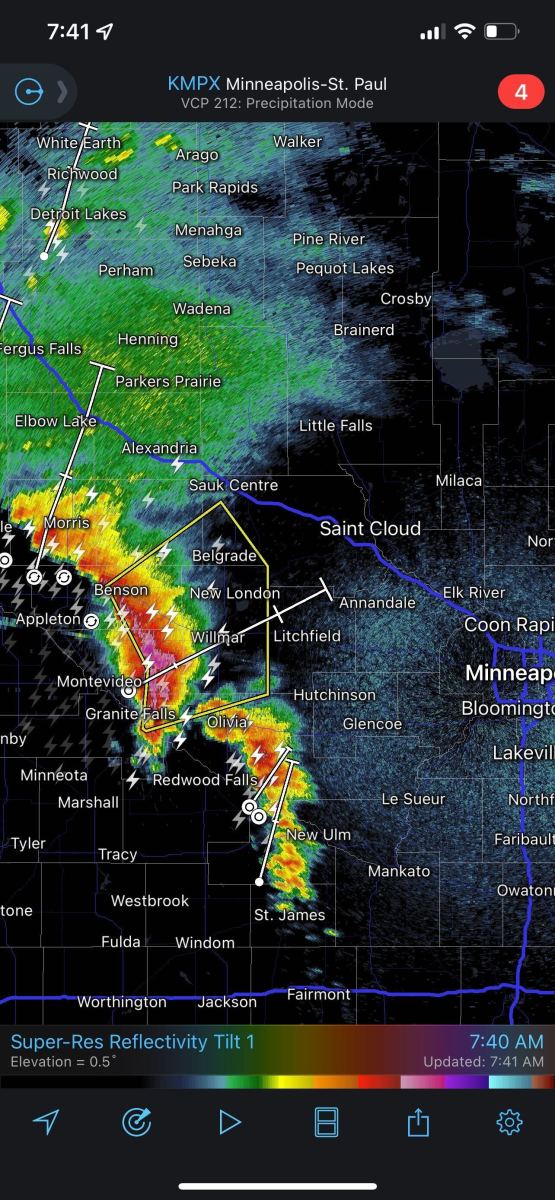The image depicts a weather map with a predominantly dark black background. Various regions on the map are highlighted in vivid colors, each indicating different weather conditions. Bright green areas contrast with blue regions, while the lower part of the map features zones colored in yellow, red, and even pink, suggesting varying intensities of weather activity. A notable city, St. Cloud, is labeled with a long blue line trailing from the upper left corner to the bottom right. The major city of Minneapolis is also visible. Towards the bottom, the phrase "Super Res Reflectivity Tilt 1" is displayed. A rainbow-colored legend runs horizontally across the bottom, displaying a spectrum of colors: green, yellow, orange, red, pink, purple, and blue. The timestamp on the map shows 7:40 a.m. with an update at 7:41 a.m. At the top of the image, the text "KMPX" appears in blue, alongside "Minneapolis-St. Paul" and the number "4" in a red circle.